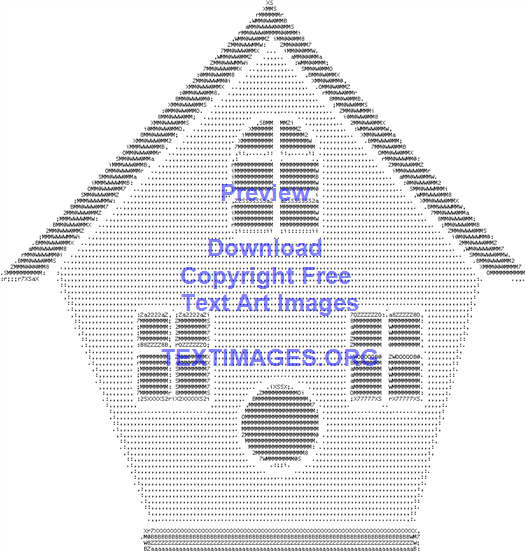This image is a computer-generated, text-based graphic of a birdhouse. The birdhouse is intricately designed using text characters, giving it a pixelated, typographical feel. The overall structure features a darker, blackish triangular roof and a lighter, hexagonal body. The birdhouse includes three windows: the top window is segmented into six parts, and the two lower windows are each divided into four sections. There's also a small circular hole near the bottom for birds to enter and exit. The birdhouse sits on a base, which is highlighted in purple. Prominently displayed in bright blue text, the foreground reads "Preview, download copyright-free text art images, textimages.org."